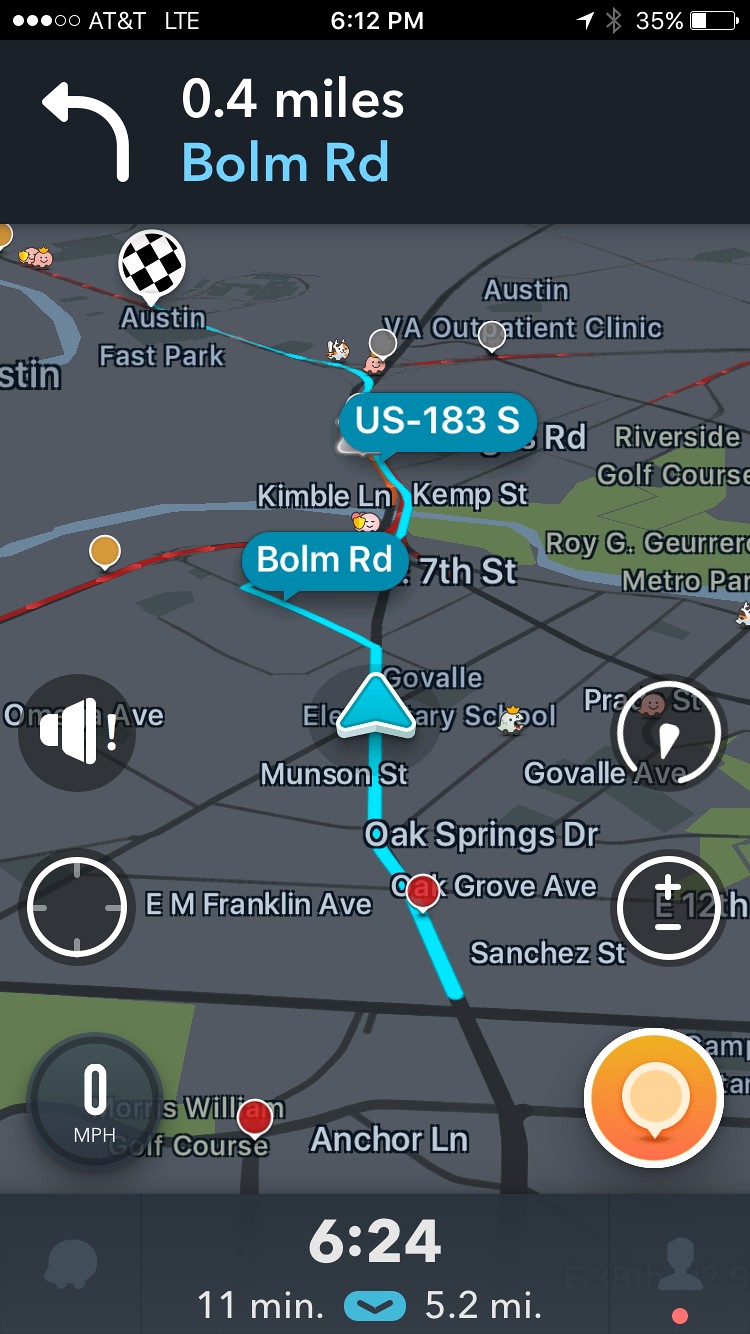A detailed screenshot of a smartphone map application shows a navigation interface with a curved white arrow at the top, indicating a left turn in 0.4 miles onto Bohm Road, which is highlighted in blue. The current route displays the vehicle's position on US 183 South, clearly marked by an arrow. Surrounding streets, such as Anchor Lane, Franklin Avenue, Sanchez Street, Grove Avenue, Oak Springs Drive, Munson Street, Govaville Avenue, and 7th Street, are visible. Austin Fast Park, potentially a go-kart or race track, is labeled on the map, alongside other landmarks like Riverside Golf Course and Roy G. Guerrero Metro Park, both situated on the screenshot's right side. The time shown is 6:24, with an estimated 11 minutes remaining to reach the destination.